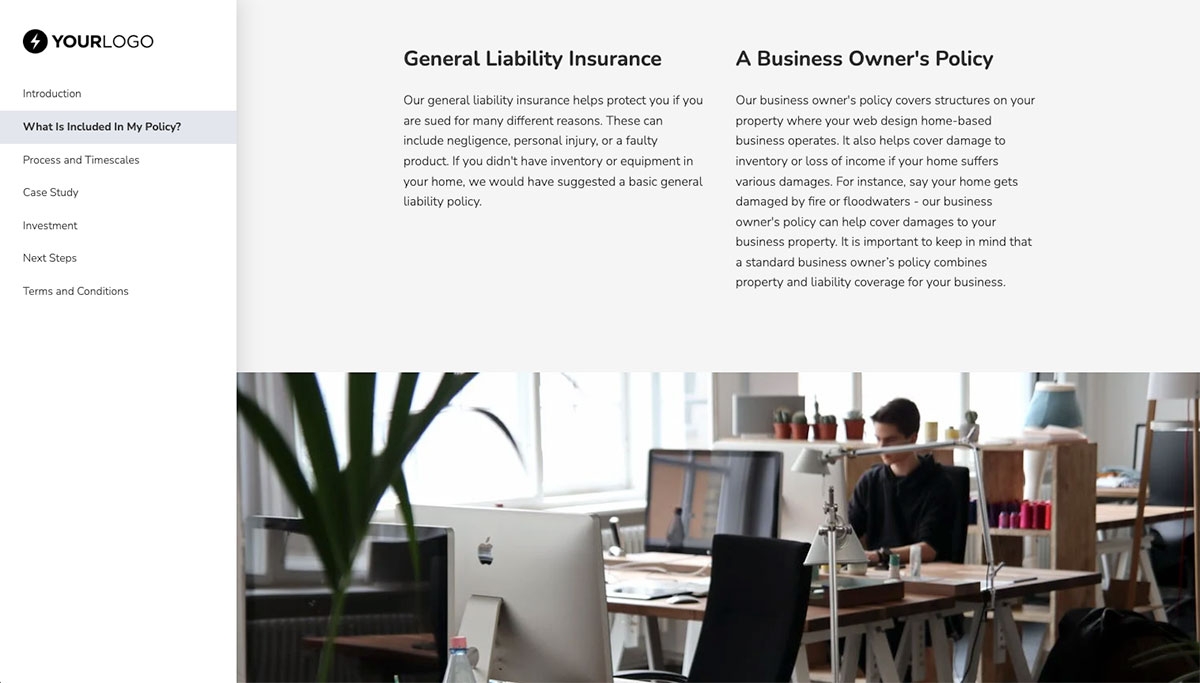This image appears to be a screenshot from a website displaying a comprehensive template for building websites, showcasing various sections related to business insurance policies. The layout includes a logo positioned on the left-hand side, and a detailed navigation panel on the left featuring a column with multiple sections such as "Introduction," "What's Included in My Policy" (highlighted in grey and currently selected), "Prices and Timetables," "Case Study," "Investment," "Next Steps," and "Terms and Conditions."

To the right of the navigation panel, detailed text outlines the specifics of each section. The highlighted section, "What's Included in My Policy," describes two core policies:

1. **General Liability Insurance:** This section explains that the general liability insurance covers legal issues such as negligence, personal injury, or faulty products. It notes that for home-based businesses without inventory or equipment, a basic general liability policy would be recommended.

2. **Business Owner's Policy:** This policy includes coverage for structures on the property used by the home-based web design business, and it extends to inventory damage or loss of income due to residential damages like fire or floodwaters. The policy combines property and liability coverage, vital for protecting business assets.

Below this textual information, there's an image of a man seated at a desk in a professional, modern-looking workspace. The man is positioned behind a metallic-framed screen, with his back to the viewer. The background includes a window, a plant, several tables, and lamps, creating a well-lit, organized office environment.